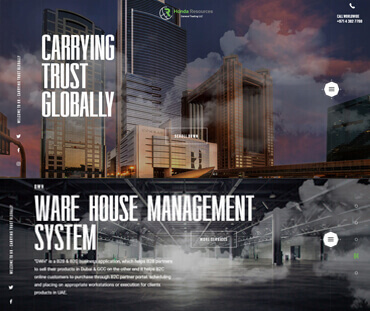A blurred printout shows what appears to be an advertisement with a mix of bold, vibrant elements and various text sections. Dominating the top left, bold words declare "Carrying Trust Globally," situated just above the phrase "Warehouse Management System." The background features a striking collage of blue, tan, and grey hues, with cloud formations against a dark sky, lending an atmospheric depth to the scene. This printout, which gives the impression of a promotional postcard, is filled with marketing materials though the precise messages are obscured. 

At the bottom, below the "Warehouse Management System," there is additional text that is unfortunately illegible due to blurring. Two round, white spots appear on the right side, adding to the visual elements. There are highlighted green segments, drawing attention to specific areas, alongside additional text aligned on the left side. The very top right corner includes an icon resembling a phone, complete with contact information likely meant for international audiences. The landscape in the backdrop is marked by tall, tan commercial office buildings, reinforcing the business-oriented theme. Finally, three dots are positioned to the left, just above the "Warehouse Management System," possibly indicating a menu or further details.